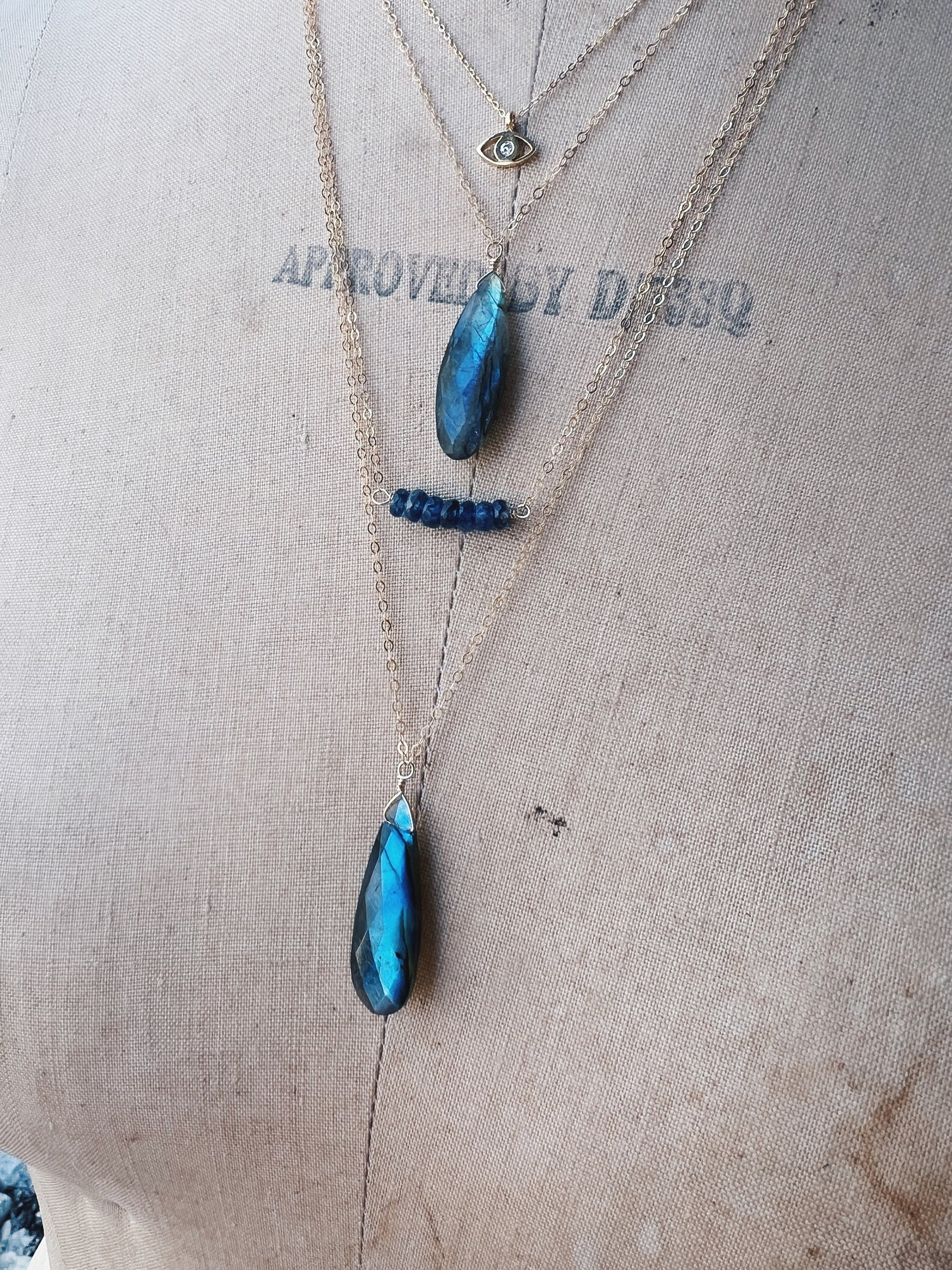The image showcases a tarnished, aged mannequin draped in a stained, brownish-white fabric, displaying a delicate silver necklace. The necklace features a vibrant, marbling turquoise gemstone that glimmers, reflecting various shades of turquoise and navy blue depending on the light. From the silver chain hangs an eye-shaped charm adorned with teardrop-shaped blue jewels, enhancing the necklace's elegant appeal. Below this charm, additional blue jewels, some reminiscent of dragonfly wings with glimmering, reflective surfaces, are attached. The old mannequin bears a faint, partially obscured stamp that reads "approved by something three three Q," adding to the vintage aura of the display.